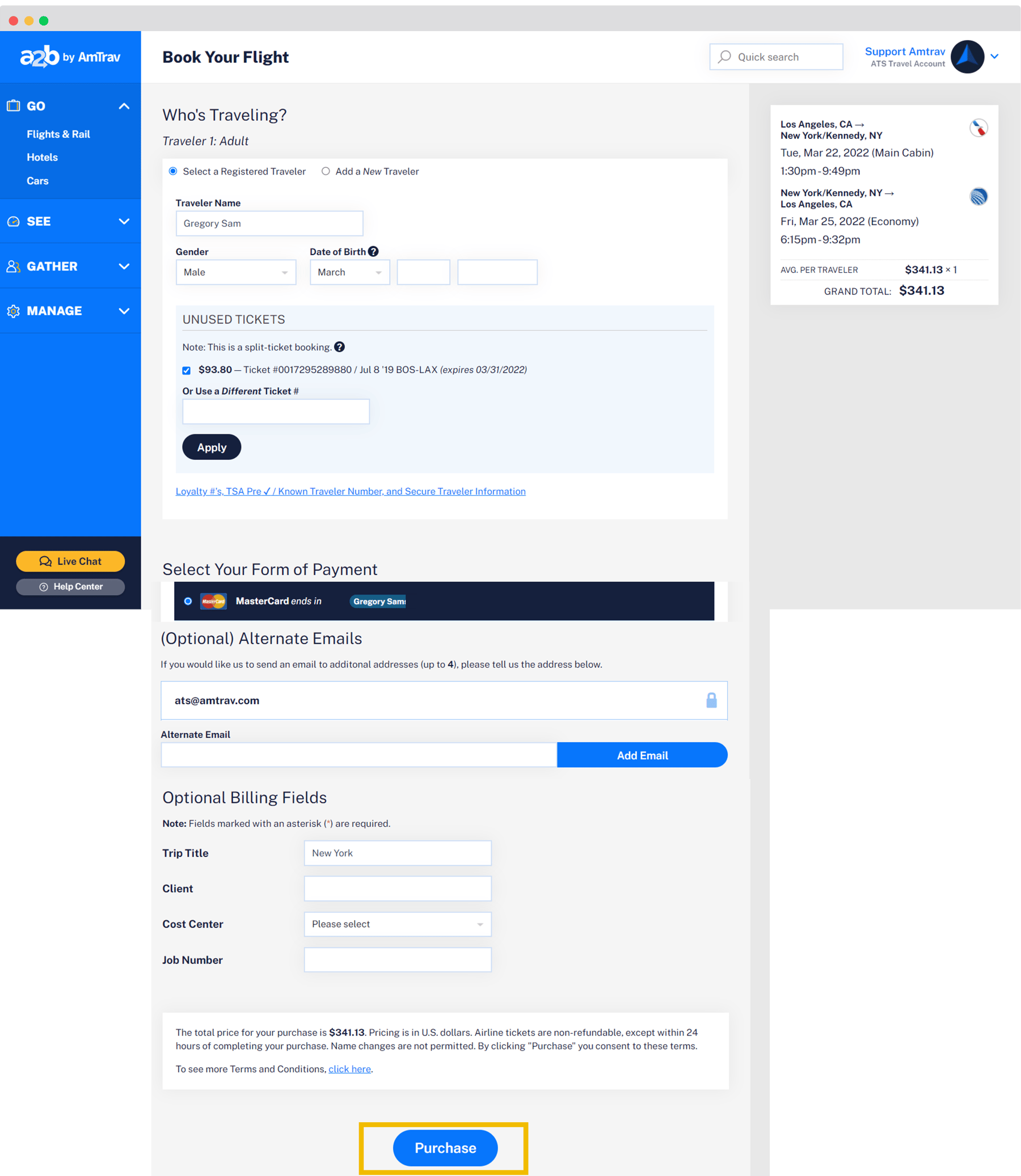This is a screenshot of the AMTRAV flight booking website interface. On the left side, there is a vertical, blue navigation bar with options such as "A to B by AMTRAV," "Go," "Flights and Rail," "Hotel," "Cars," "See," "Gather," "Manage," "Live Chat," and "Help Center."

At the center of the page, under the heading "Book Your Flight," the section "Who's Traveling?" is displayed with one registered traveler. Currently, "Traveler One" is identified as Gregory Sam, male, born in March. The form also provides options to select a registered traveler or add a new one. The current traveler details include Gregory Sam's name, gender (male), and date of birth (March), with two other fields remaining empty.

Below the traveler's information, there is a note about unused tickets, specifically mentioning that this is a "split ticket booking." Details include a ticket number (9380), booking date (July 8th, 19), route (BOS to LAX), and expiration date (03/31/2022). There is also an option to use a different ticket number, alongside an "Apply" button.

Further down, the form requires selecting the payment method, which here shows "MasterCard" presumably highlighted as the chosen option. The section for adding optional alternative emails includes one sample email (ATS@AMTRAV.com) with instructions to enter up to three additional email addresses to receive booking details.

This detailed description captures the structure and content of the AMTRAV flight booking interface as illustrated in the caption provided.